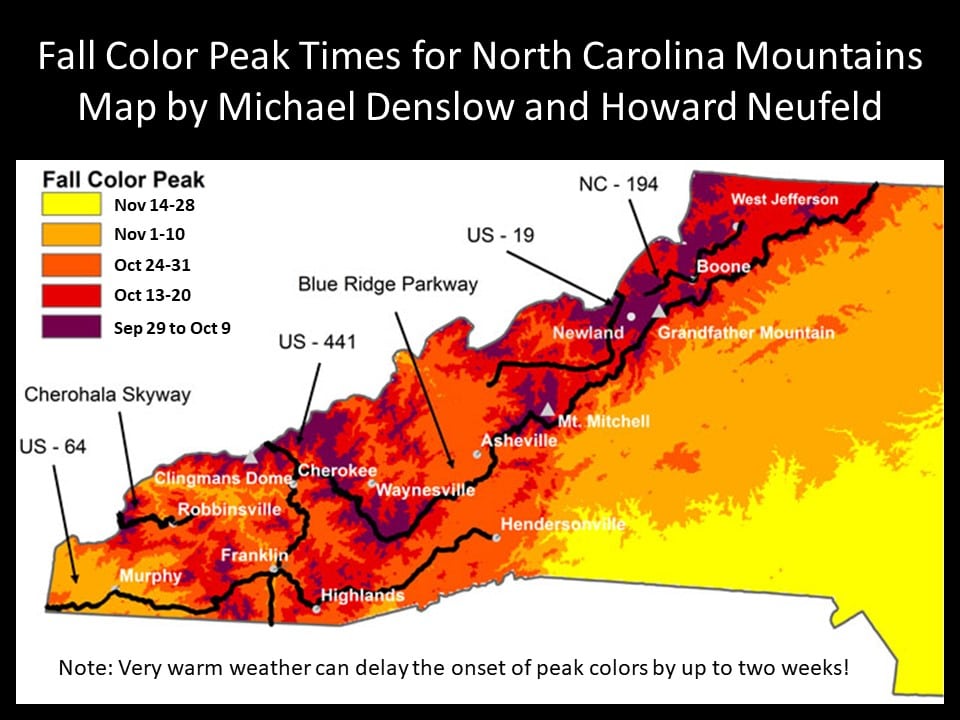The image is a detailed heat map depicting the fall color peak times for the North Carolina mountains, created by Michael Denslow and Howard Neufeld. The top of the image contains a black banner with the title, "Fall Color Peak Times for North Carolina Mountains," in white text. The peak times are color-coded: yellow (Nov 14th-28th), orange (Nov 1st-10th), deep orange (Oct 24th-31st), red (Oct 13th-20th), and burgundy (Sept 29th-Oct 9th). The heat map emerges from the right, narrows down through the center, and stops at the bottom left corner. Throughout the map, various locations and landmarks such as U.S. 64, Cherohala Skyway, Blue Ridge Parkway, Boone, Newland, Mount Mitchell, Asheville, and Waynesville are labeled. At the bottom of the image, black text notes, "Very warm weather can delay the onset of peak colors by up to two weeks." The background is white with a black border, thicker at the top.